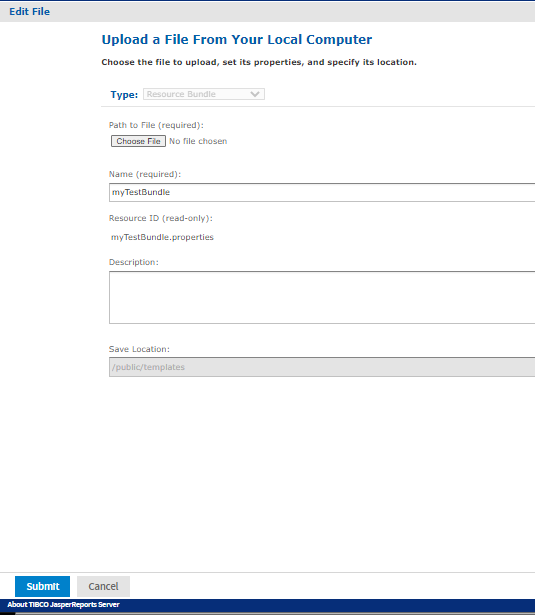The image displays a screen for uploading a file from a local computer, divided into distinct sections. At the top, there's a gray bar with the blue text "Edit File." Below that, the main white section begins with a blue header that reads "Upload a file from your local computer."

Underneath the header, there's an instruction in black text: "Choose the file to upload, set its properties, and specify its location." Following this, a labeled section appears for specifying the file type. The label "Type" is in blue, accompanied by a drop-down menu set to "Resources Bundle."

Continuing downward, there's a section labeled "Path," indicating that the path of the file is required. This section includes a "Choose File" button, followed by the text "No file chosen" when no file selection has been made.

Further down, there is a "Name" section, marked as required, featuring a textbox pre-filled with the text "my_test_bundle." Beneath this, in a read-only format, is the "Resource ID," followed by the text "my_test_bundle_properties."

Next is the "Description" section, containing an empty textbox for user input. Below that is the "Save Location" field, with the textbox pre-filled with "/public/templates."

Finally, at the bottom of the screen, there are two buttons: a blue "Submit" button and a gray "Cancel" button.